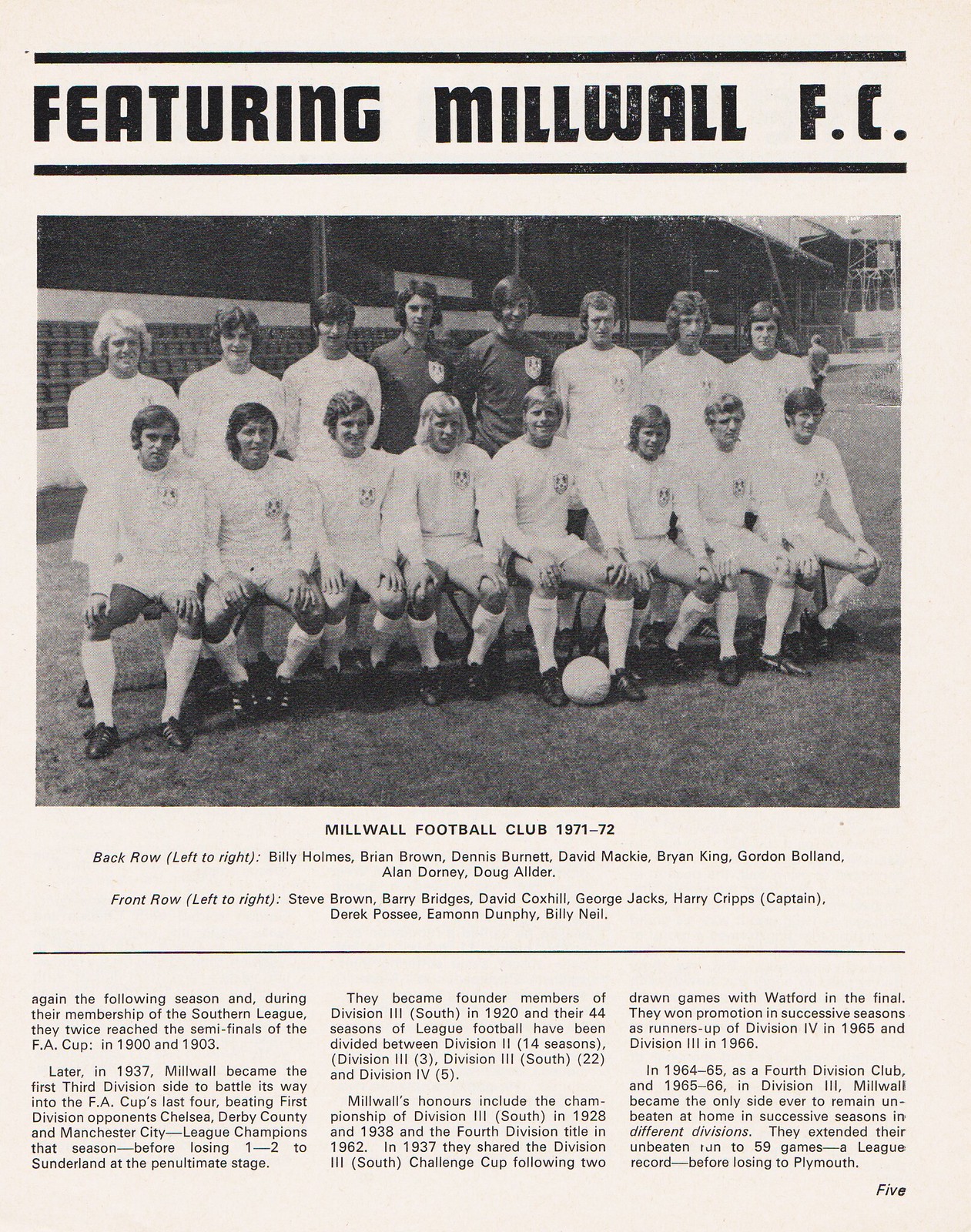The image is a black-and-white photograph from a possibly worn and dated newspaper clipping or football program page, featuring the Millwall Football Club from the 1971-1972 season. The text at the top reads "Featuring Millwall FC, Millwall Football Club." The photograph depicts a male soccer team arranged in two rows on a grassy field. The first row consists of players sitting down with one player holding a football between his feet, while the second row has players standing up and smiling. Most players are in white uniforms, except for two in the middle of the back row who are wearing darker tops. Beneath the picture, the caption reads "Millwall Football Club, 1971-1972." The names of the players, listed from left to right, include: 
Back row: Billy Holmes, Brian Brown, Dennis Burnett, David Mackey, Brian King, Gordon Boland, Alan Dorney, Doug Alder.
Front row: Stephen Brown, Barry Bridges, David Coxhill, George Jacks, Harry Cripps (captain), Derek Posse, Eamon Dunphy, Billy Neal.
Additionally, there is a text section underneath the caption that describes the history of the football club and recounts their victories and losses during that period.